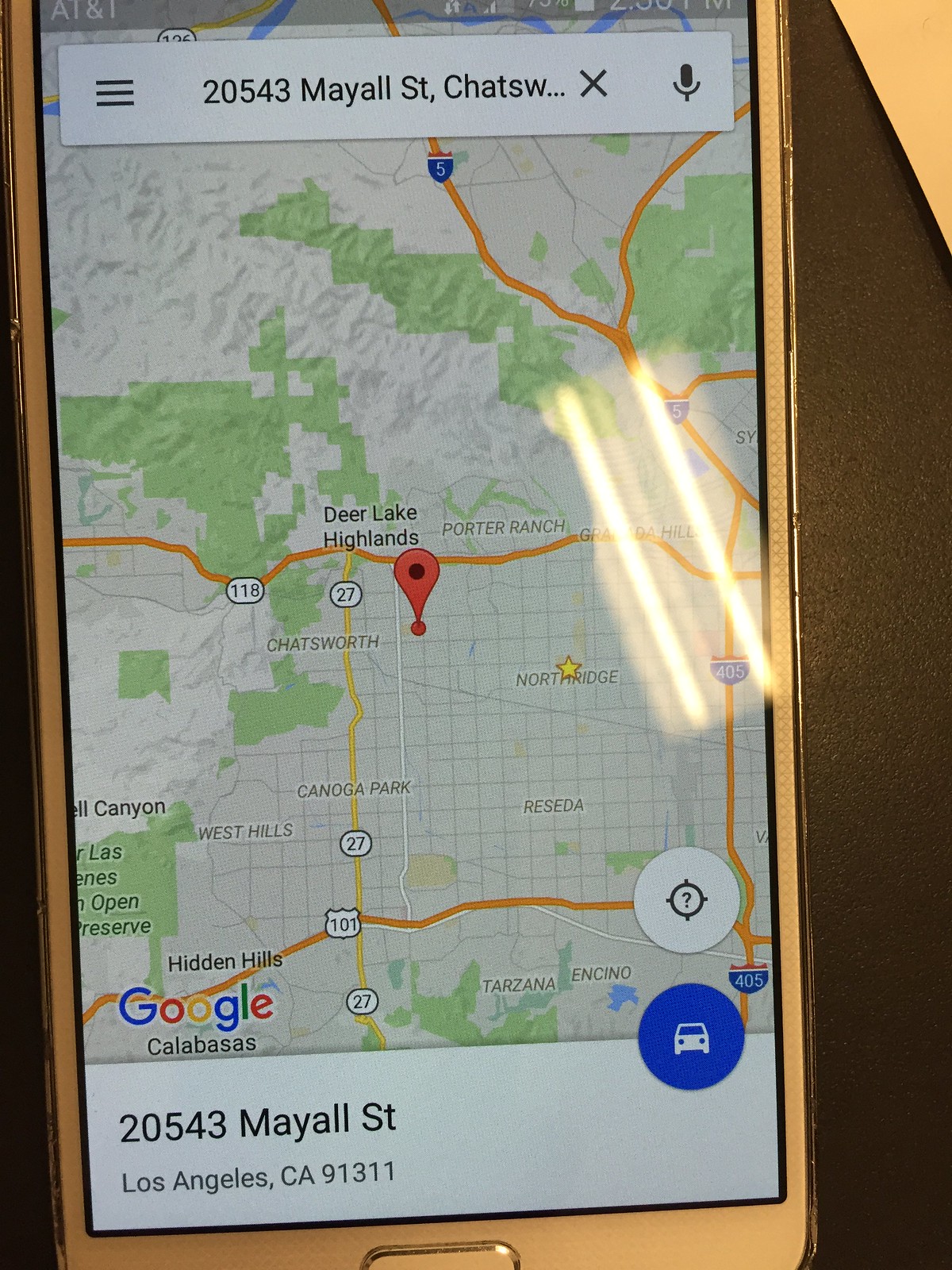The image captures a smartphone displaying a navigational map. The device, branded with the AT&T icon on the top, is currently searching for the address "20543 May Yall Street, Los Angeles, CA 91311." Part of the address search visible at the top reads "20543 May Yall Street, CHAT..." which is truncated, followed by an "X" to clear the search and a microphone icon for voice search input. The search results highlight Deer Lake Highlands, with the map displaying surrounding roads and streets.

Below the search bar, the full address is clearly printed as "20543 May Yall Street, Los Angeles, CA 91311." Adjacent to this are two icons: the first is a car representing GPS directions, and the second is a bullseye-like symbol, possibly for dropping pins. The top interface of the phone, which includes standard indicators like the time and battery percentage, is partially visible but cut off. The overall map view mainly displays the query area, emphasizing its geographical layout and connected routes.